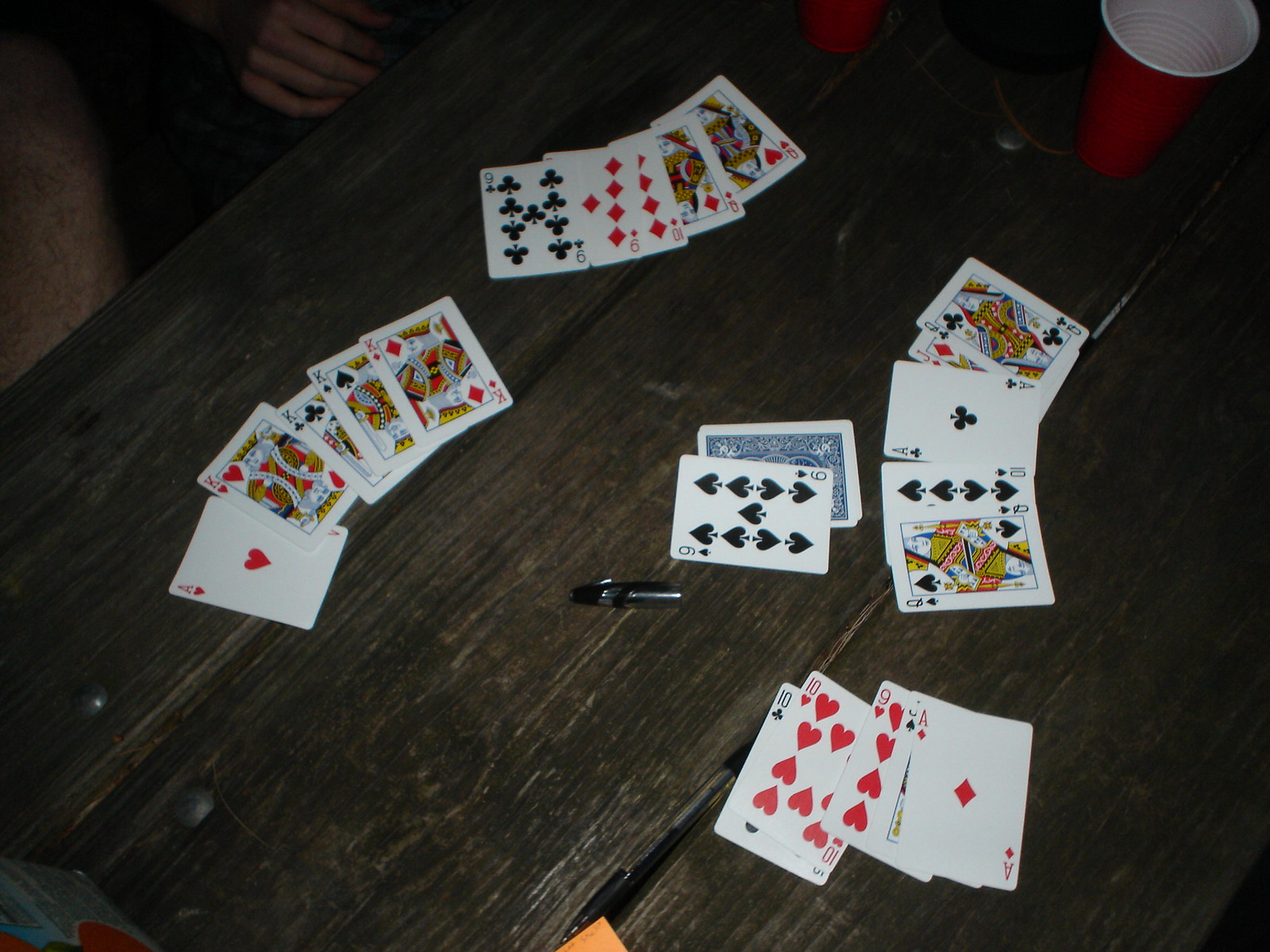Captured in a high-angle photographic style, this nocturnal scene showcases a dark brown wooden table illuminated under soft lighting. Scattered across the table are playing cards arranged in four distinct hands, each consisting of four to five cards laid face-up. The familiar symbols and numbering of a standard deck are clearly visible. Prominently, a black-capped pen with transparent elements lies next to the nine of spades, which rests atop a small deck of facedown cards centrally positioned on the table. Two red cups are situated in the top right corner, suggesting a casual, social atmosphere. In the top left, a faintly lit Caucasian hand and leg are barely discernible against the shadows, adding a sense of human presence to the engaging tableau.